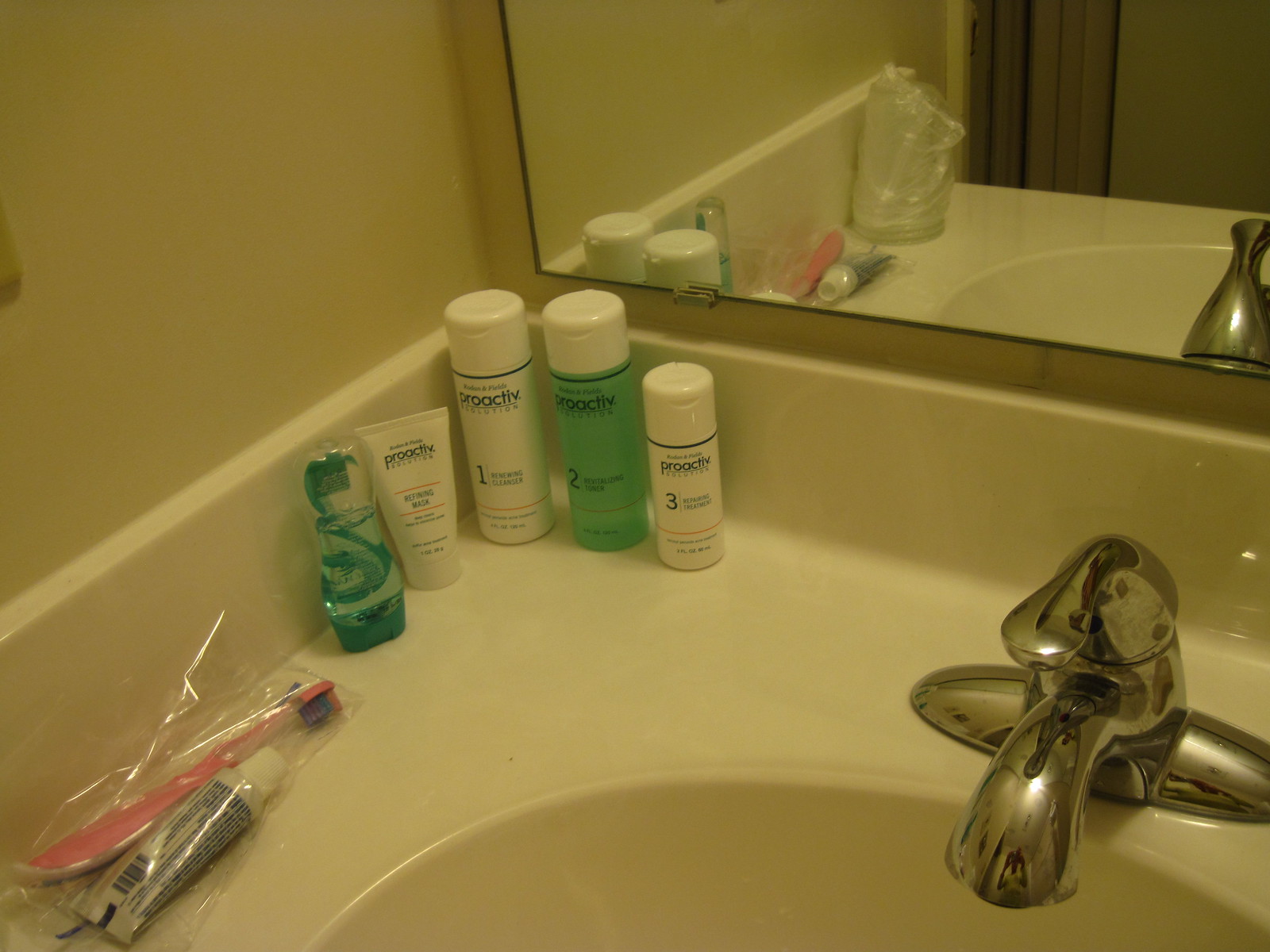The photograph depicts a corner of a bathroom sink area, likely in a hotel room, as indicated by the travel-size toiletries. The background wall is a basic beige or cream white color. The sink itself is white porcelain with a marble-esque finish, and features a chrome faucet with a single lever to adjust water temperature and pressure, positioned near the bottom right of the image. In the corner of the sink, there is a small transparent plastic bag containing a pink toothbrush and a tube of white toothpaste adorned with blue writing.

Five bottles of ProActive Solution, an over-the-counter acne treatment, are also visible. These bottles are slender and bullet-shaped, with variations in design and labeling. The bottle furthest to the right is white with blue designs and labeled "ProActive 3." The next bottle, green with a white cap, features the number "2." The middle bottle is white with dark green text and marked with the number "1." The fourth bottle, second from the left, also bears similar writing but has a functioning mask on the center. The final bottle on the far left is transparent and filled with a green substance.

A mirror on the right side of the image reflects the toothbrush, toothpaste, and bottles. Additionally, three plastic-wrapped cups can be seen reflected in the mirror, further indicating a hotel setting.